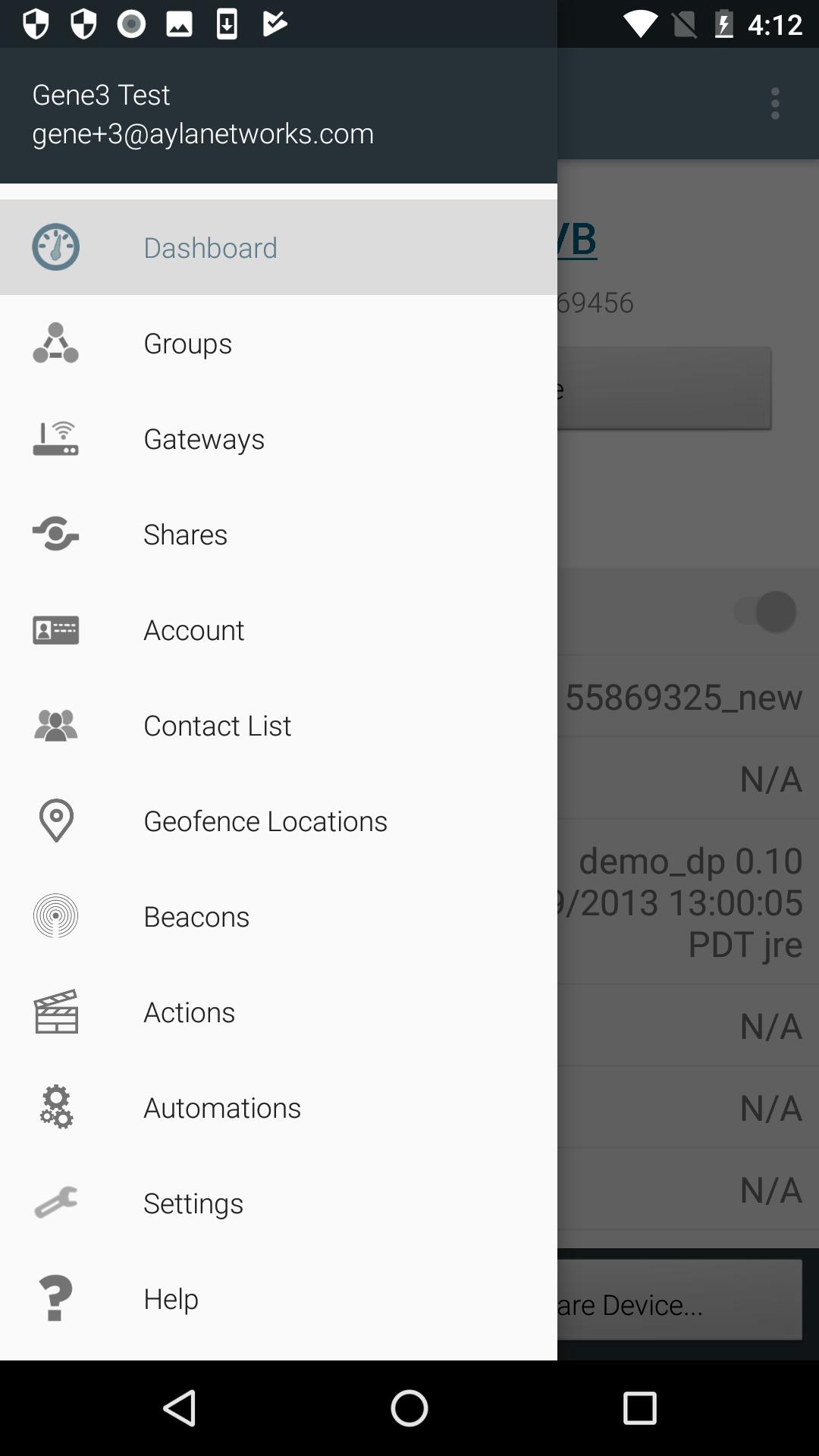A detailed screenshot of an Android smartphone displays several notable elements. In the top-left corner, six icons can be observed, followed by a Wi-Fi icon towards the center-right. The Wi-Fi icon appears as a small white box with a black diagonal line. Adjacent to it, a low battery symbol containing a white lightning bolt indicates that the device is charging. The current time shown is 4:12 PM, with most icons appearing in white color for clarity.

Beneath this status bar, a menu is open on a page with a dark gray background and white text. The text at the top reads "gene three tests," followed by "gene++3 at Ayla and et works comm." To the left part of the screen, a white background section is displayed where a gray-highlighted item, labeled "Dashboard" in blue text, is prominently featured.

This sidebar menu has a vertical list of icons and text describing various sections. The sections listed, in order, are: Dashboard, Groups, Gateways, Shares, Account, Contact List, Geofence, Locations, Beacons, Actions, Automations, Settings, and Help. Each section name is supported by a relevant icon, although the description mainly focuses on the text labels for clarity.